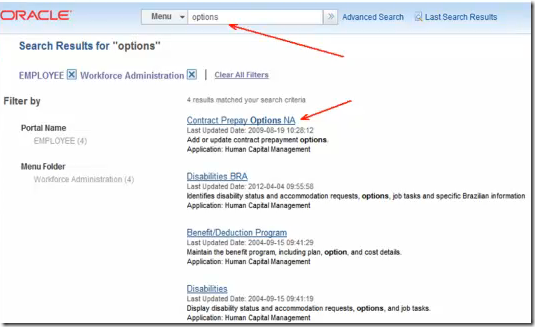**Detailed Caption:**

The website interface features a light blue header at the top. In the top right corner, the word "Oracle" is prominently displayed in red. Below this, a black text "Menu" is visible inside a menu box. Adjacent to this is a search box outlined in gray with a white interior, containing the black text "Options". A red arrow points towards the lower outline of this search box for reasons unspecified.

To the left, beneath the light blue header, the page background transitions into white. Blue text reads "Advanced Search" followed by "Last Search Results". On the left, the blue text "Search results for" is displayed, with the keyword "options" highlighted in black quotations.

Further down, the search results are listed with specific details:
- In purple, the term "Employee" appears alongside a blue 'X' icon.
- Another item, "Workforce Administration", also in purple with a corresponding blue 'X'.
- Below these results, an underlined purple text reads "Clear Filters".

The section "Filter By" in black is followed by "Portal Name: Employee" and "Menu Folder". For instance, under "Workforce Administration", there is an entry marked "In four". In blue, the text "Contract Prepaid Options" is shown with another inexplicable red arrow pointing towards it.

Continuing down the page, black text details the "Last Update: 2009-05-19, 10:28:12", which reads, "Adult Update - Contract Prepayment Options Application... Human Capital Management". Following this, more items appear:
- In blue, "Disabilities VRM".
- Underlined black text reads "Last Updated 2012-04-04-09... 55... 58 - Identifies Disability Status and Accommodation Request".
- A list of options indicates specific applications like "Jobs have specific Brazilian information application" and "Human Capital Management".
- In blue, "Benefits and Deduction Program" and "Disabilities" are also listed.